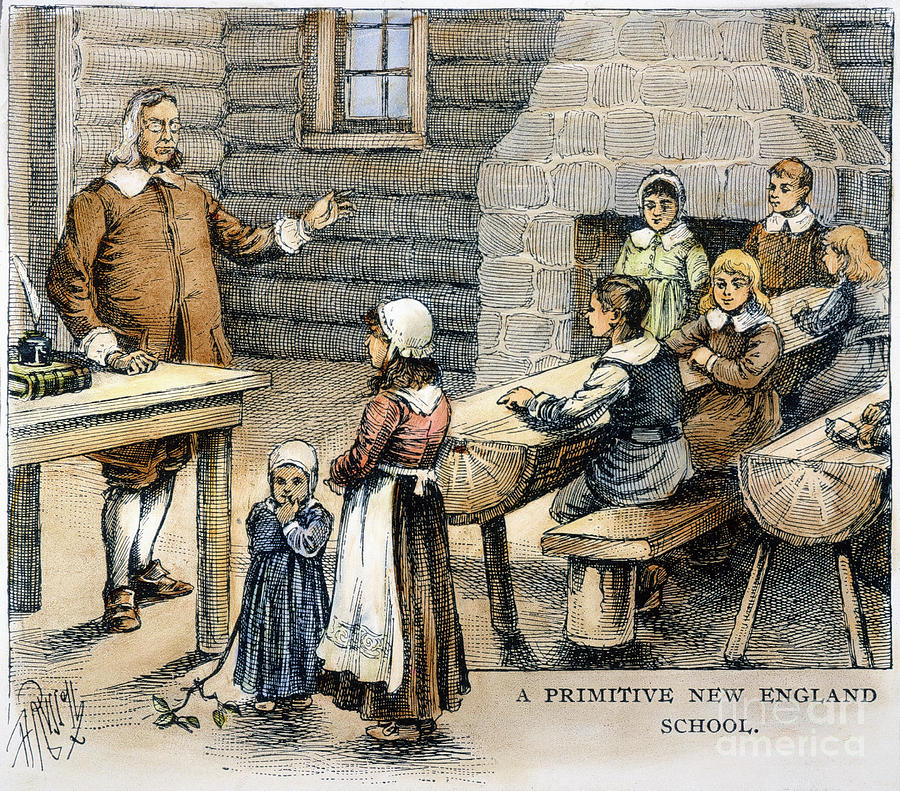The image depicts a detailed illustration of a primitive New England school, reminiscent of colonial times. The scene is set within a log-cabin-style schoolhouse, characterized by its log walls and prominent stone fireplace. At the front of the class stands a teacher, an older man with white hair styled similarly to Benjamin Franklin, wearing glasses, a brown coat, white tights, and 1700s-style buckle shoes. He is gesturing with one hand raised while the other rests on a desk adorned with a green book, an ink blotter, and a feather quill.

The children, dressed in various colonial-era clothing colors such as blue, brown, green, and red, sit on benches made from halved logs, used as desks. Some of the girls wear dresses and bonnets. The students appear attentive, focused on their teacher's instruction. The overall artwork, likely a lithograph or pen-and-ink illustration, captures the essence of a rustic, early American educational setting, as indicated by the label, "a primitive New England school," visible in the bottom right corner of the image.